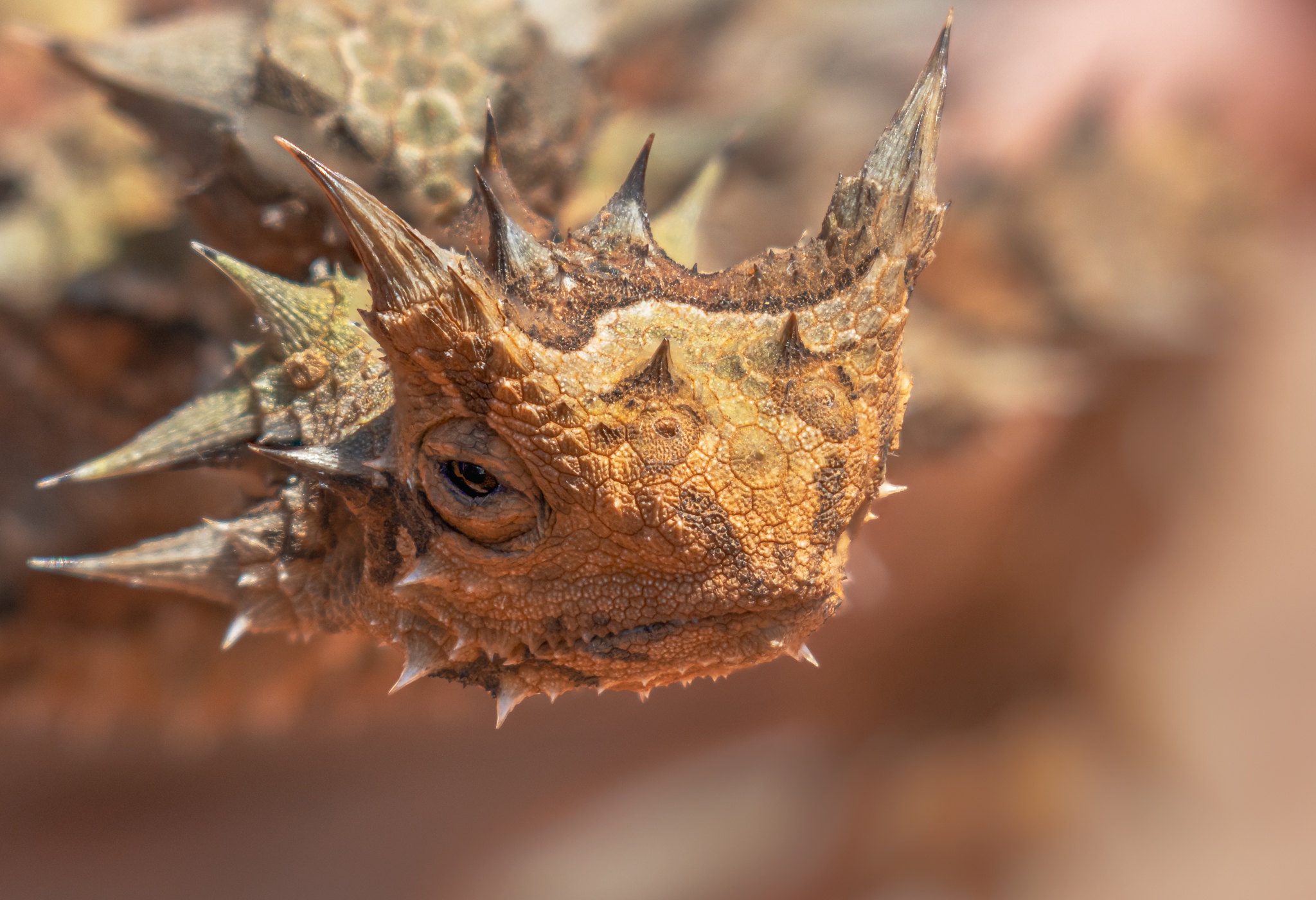This is a detailed close-up color photograph of the head of a thorny devil lizard, a species native to Australia. The creature's face, sharply in focus against a blurry backdrop of red, brown, and yellow hues, is predominantly patterned in shades of light and dark brown, with touches of green. The lizard's head is characterized by a pointy, spiked appearance with prominent horns on either side where its ears would be, and additional spikes running down its neckline and body. The facial spikes and some on its lower body are tipped in white, resembling tiny wooden thorns. Only the right eye is visible in the image, featuring a black pupil encircled by a light brown iris, set within wide eye sockets and surrounded by a circular indentation. The overall setting appears to be daytime.